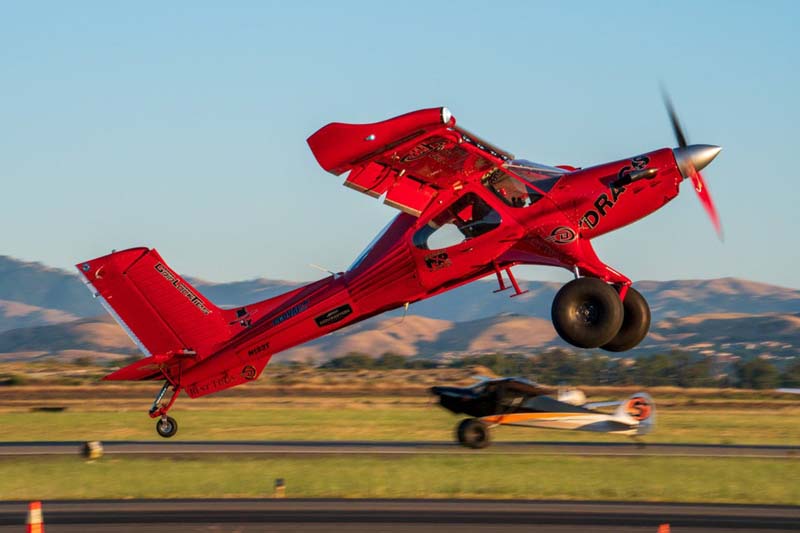The photograph showcases a dynamic scene of two airplanes, with the focal point being a bright red, fire-engine red single-prop airplane prominently displayed in the foreground. This well-maintained, single-wing plane is caught in the moment of ascent, having just taken off from the runway. Its nose is pointed diagonally upwards towards the top right corner of the image, while the tail, equipped with a small rudder wheel, is closer to the ground. The plane's large black wheels are visible and off the ground, underscoring its recent departure. There appears to be something written on the side of the plane, possibly "DRAGS."

In the background, there is a second airplane situated on the runway. This airplane features a striking black color with orange stripes and bears an 'S' on its back wing. The second plane's activity is ambiguous, as it may be either landing or taxiing. The entire scene is set against a backdrop of expansive grassy fields and distant hills or mountains that take on a bluish-gray tone, under a clear blue sky. The overall image exudes a sense of motion, energy, and vitality, capturing the excitement of aviation against a scenic landscape.